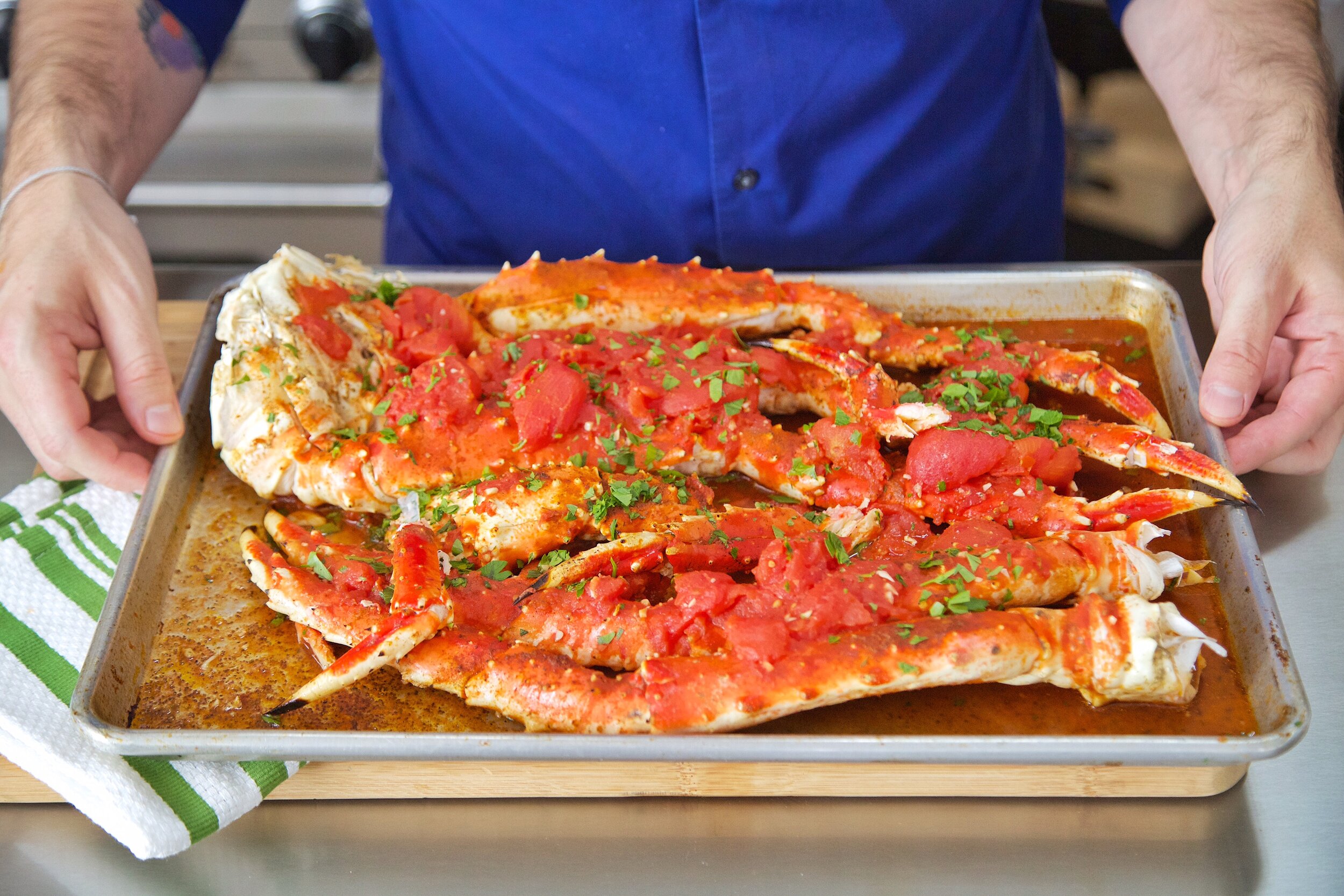A man, wearing a dark blue short-sleeved button-down shirt, holds a metal baking tray filled with cooked crab legs. The crab legs are garnished with diced tomatoes or red peppers and adorned with small green leaves. The tray, which shows signs of prior use, sits on a light-colored wooden cutting board. A white cloth with green stripes lies beneath the left side of the tray, which also holds a brown sauce at the bottom, indicating the crab legs have been baked. The man has a bracelet on his right wrist and a visible tattoo in shades of purple and red on his right forearm. The overall scene suggests a well-prepared seafood dish ready to be served.